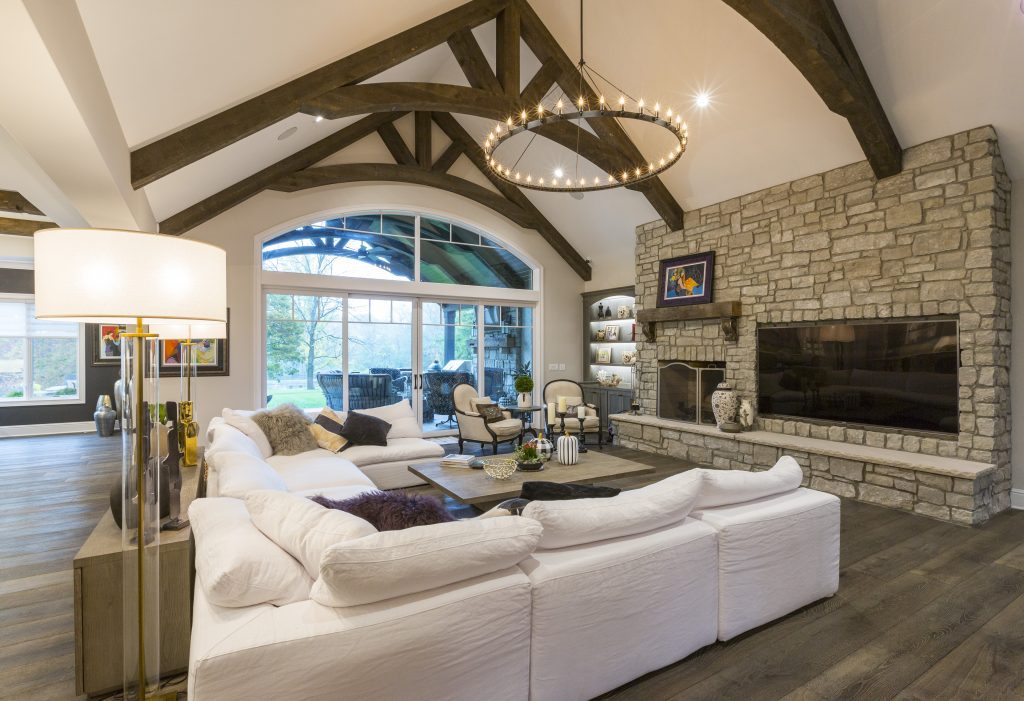This image captures a beautifully modern and stylish living room in a new building. The spacious room is meticulously clean and neatly arranged, featuring a prominent stone fireplace with a wooden mantel. A large flat-screen TV is mounted on the wall to the right of the fireplace, while a triangular roof with exposed curved wooden beams adds architectural interest to the space. Hanging from the ceiling is an eye-catching circular chandelier with multiple lights, contributing to the room’s bright and inviting atmosphere.

The seating arrangement includes a large, white sectional couch configured in a double L-shape that extends to three sides of the room, centered around a square coffee table. Two identical pole lamps with white shades are positioned on either side of the couch. The room’s parquet wooden floor enhances its warm aesthetic.

Towards the back of the room, large windows and glass doors open up to a covered patio, where outdoor furniture invites relaxation. Inside, near the patio doors, two additional chairs and a small table create a cozy conversation area. Adding to the room’s decor, there are shelves beside the fireplace, paintings on the wall, and additional soft lights in the background.